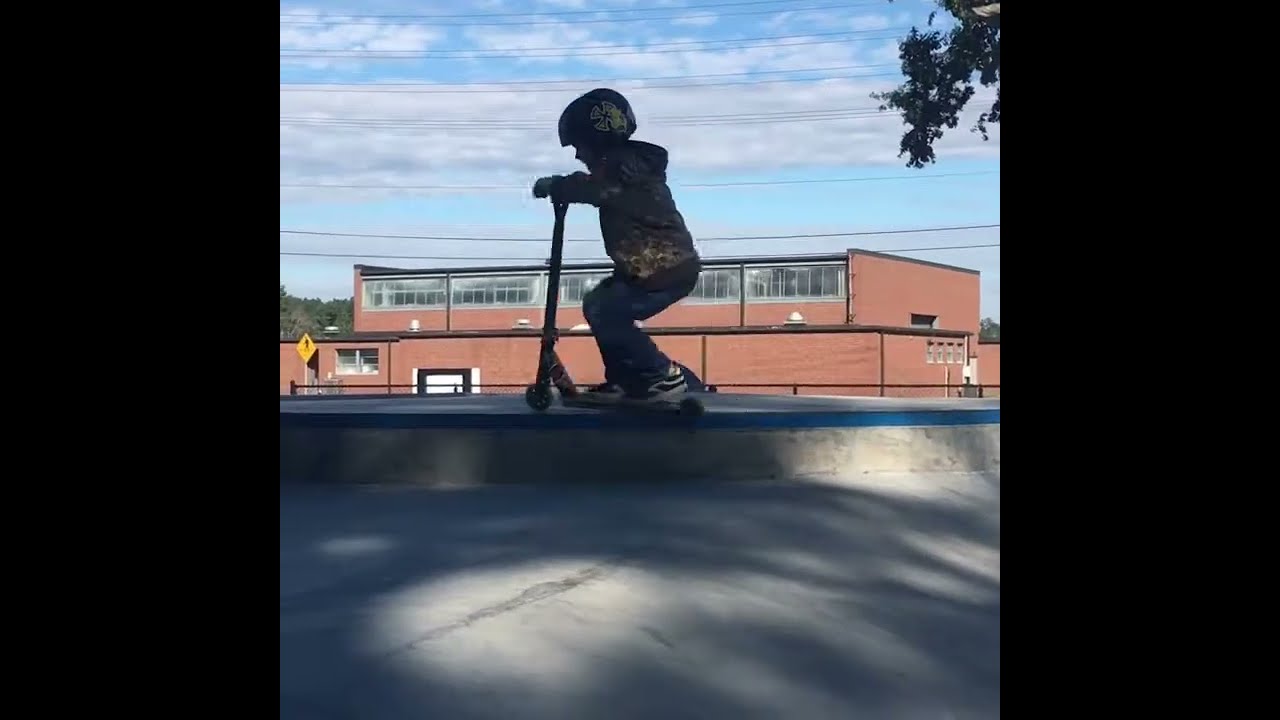In this vibrant photograph, a child wearing a helmet, hoodie, jacket, jeans, and tennis shoes is captured in silhouette while riding a scooter on an elevated section of a skateboard ramp. The setting appears to be a skateboard park. The scene is bathed in sunlight, although the child and parts of the ramp are in shadow, creating a dynamic play of light and dark. The background features a large, two-story wide brick building with many windows on the second story, suggesting it could be a school or office. The reddish-orange hue of the building contrasts with the bright blue sky and scattered white clouds above. Electrical lines stretch horizontally across the upper portion of the image. In the top right-hand corner, the silhouette of a tree branch is visible. A yellow diamond-shaped sign is positioned in the lower left-hand corner, and beyond the building, a stand of trees enhances the natural ambiance of the scene.